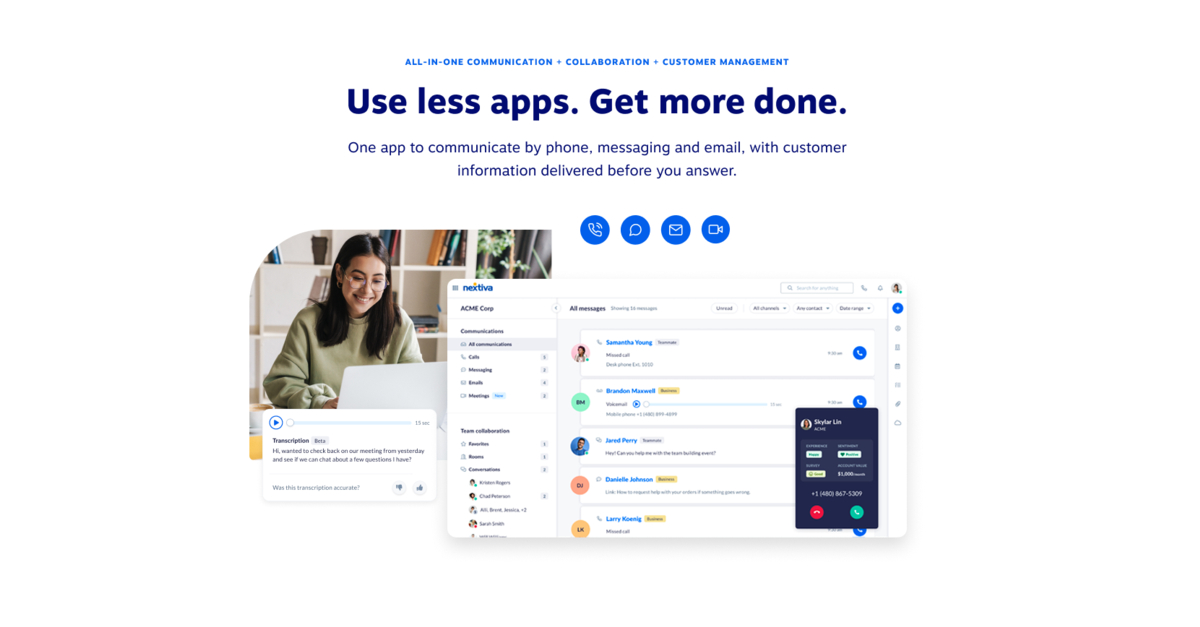The left side of the image features a woman typing on her laptop, looking downward. She is wearing a very light green, almost light gray colored sweater and has long hair. The woman is also wearing sunglasses and is smiling. At the top of the image, there is a title in dark blue font that reads, "Use less apps, get more done." Below this title, a description states, "One app to communicate by phone, messaging, and email with customer information delivered before you answer." In the bottom right-hand corner, a small, blurry webpage is displayed. The webpage, with a predominantly white background, appears to show several individuals that one can click to communicate with via text, email, video chat, or call, indicating it is a communication service.